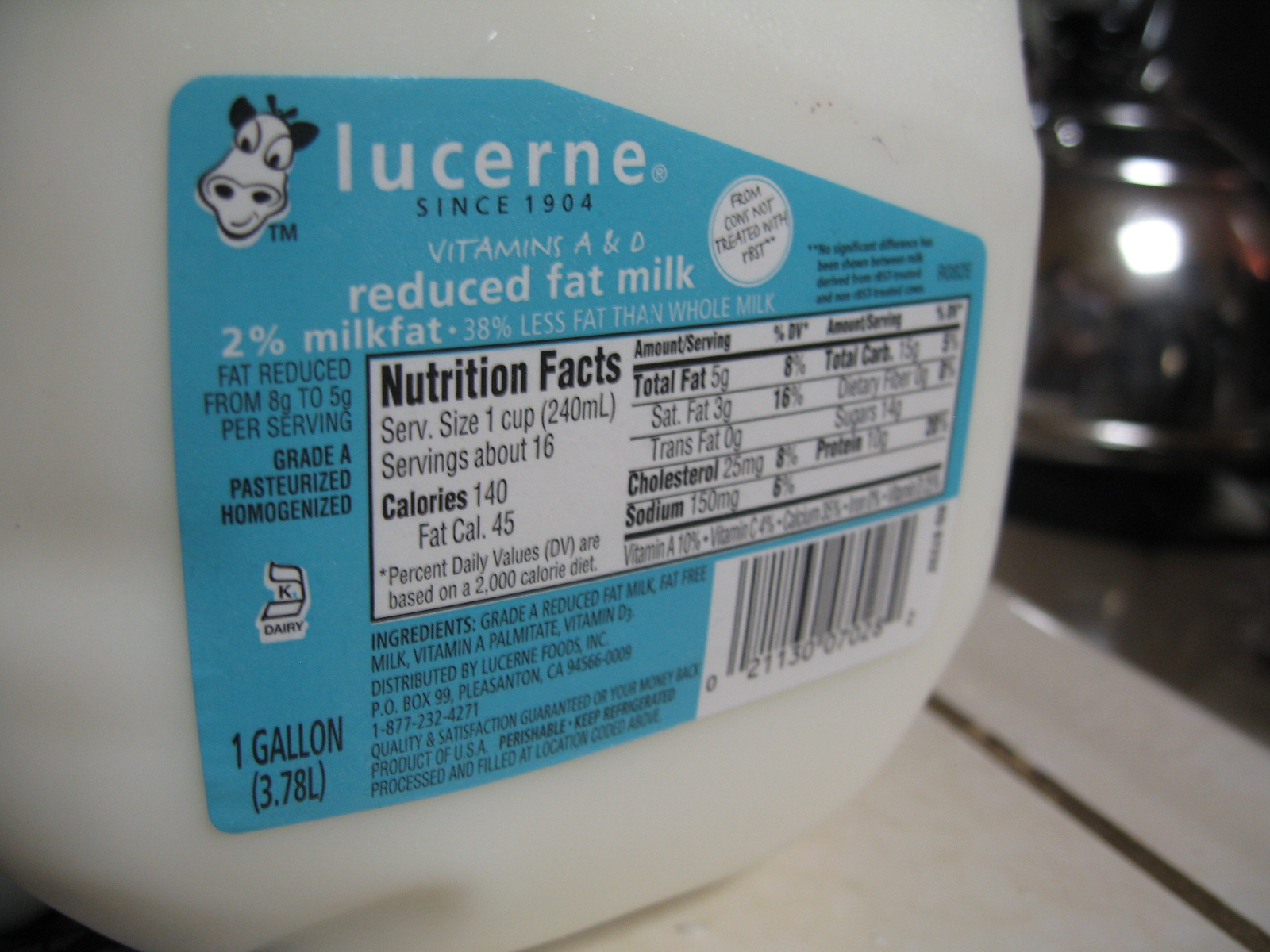This color photograph features a close-up of a plastic milk jug placed on a white surface. The jug is predominantly white with a blue label prominently displayed. The label includes a small image of a cow located at the upper left-hand corner, next to which is written "Lucerne Since 1904." Below this, larger text reads "Reduced Fat Milk, 2% Milk Fat," followed by smaller, unreadable text. On the bottom left corner of the label, it clearly states "One Gallon, 3.78 Liters." Positioned at the bottom right-hand side, a barcode is visible. Adjacent to this on the blue section of the label is a white nutritional information panel with black text detailing various nutrient amounts such as fat, cholesterol, and sodium. The ingredients list, which is printed in small black text, is located to the left of the barcode. In the background, through a window visible on the right side of the image, blurred lights and possibly a car can be seen, suggesting the photograph was taken in an interior space with some external light filtering in.